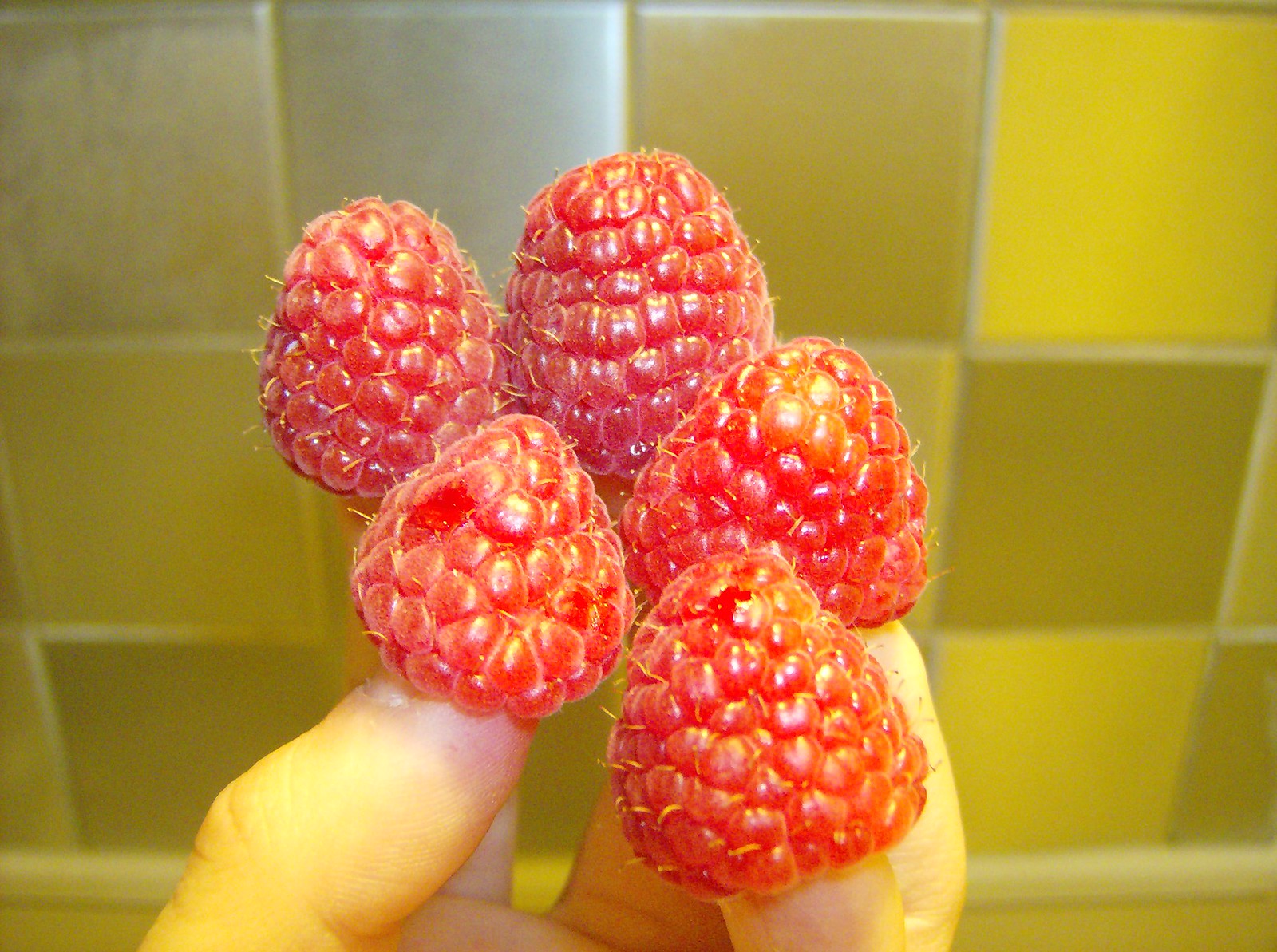This is a detailed color photograph of a right hand with one bright red raspberry perched on the tip of each finger, resembling tiny hats. There are five raspberries in total, and while most are in perfect condition, the one on the thumb is slightly dented. The fingertips, though not fully visible, are clearly holding the berries. The background features a kitchen wall tiled with alternating squares of yellow and various shades of green, separated by white grout. There’s additional light creating reflections on the raspberries, suggesting a flash was used in conjunction with the existing ambient light. A dark cream or pale green countertop is also partially visible at the bottom, adding to the indoor setting.